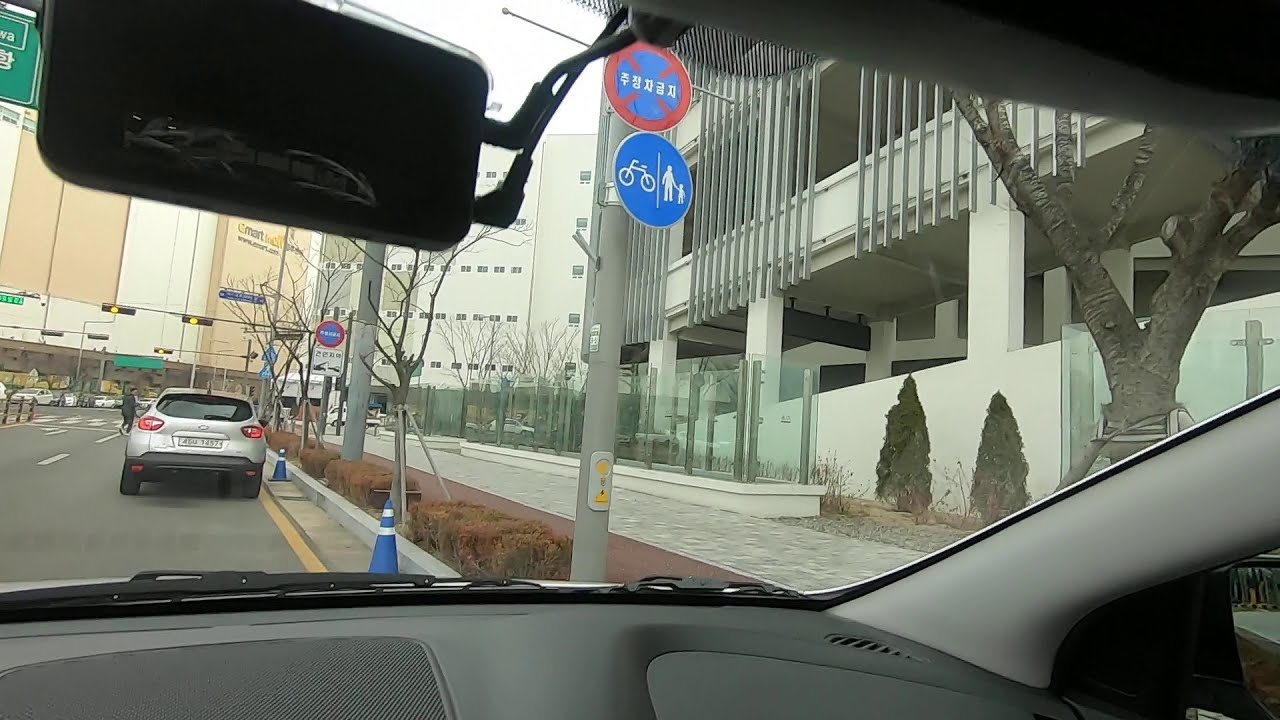The image captures the point of view from within the front seat of a car, likely parked on the side of a road in an Asian city. In the upper left corner, the rearview mirror is visible. Just ahead, slightly to the right of the car, there is a gray pole with two circular signs: the top sign is blue and red featuring Asian text, possibly indicating no parking, and the lower sign is blue with white symbols depicting a bicycle and animated figures of an adult and child. The car seems to be parked at the curb, where blue safety cones with white stripes are positioned nearby. In front of this car, there is a gray sedan, and a person is seen crossing the street. The streetlight above is yellow, suggesting a transition. On the right side of the street, a small median with bushes separates the road from a red brick sidewalk and a gray stone sidewalk. A tall building with vertical decorative bars extends out of the frame on the right side. The interior of the car features a mounted tablet device on the windshield, adjacent to the rearview mirror.